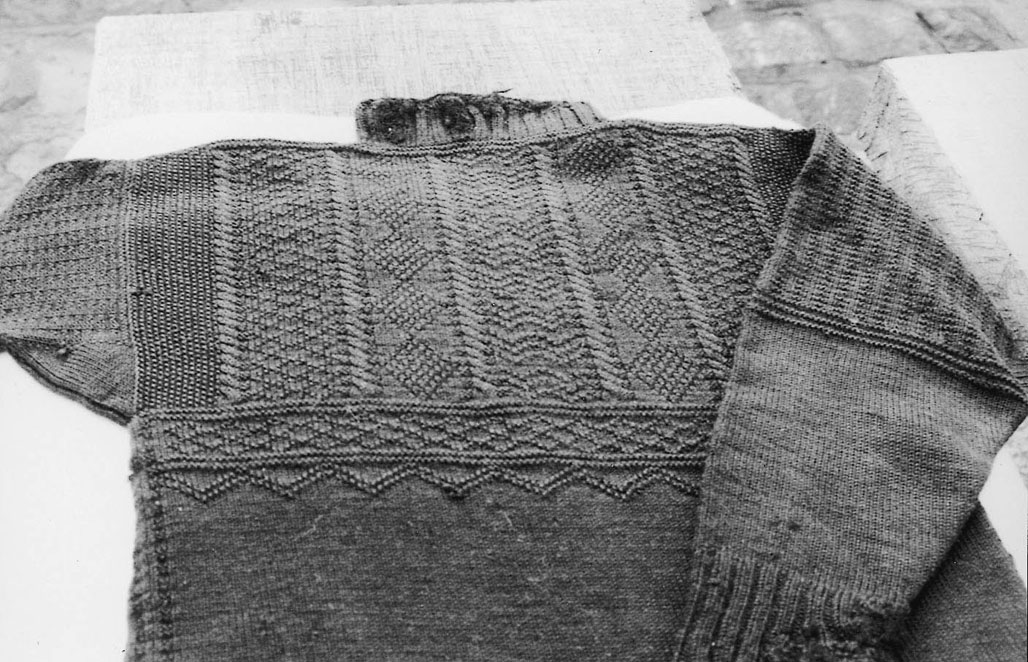This image displays a detailed view of an unfinished dark grey, knit sweater laying on a light stone ground. The sweater, possibly made of wool or cotton, features a diverse array of intricate patterns dominated by triangles, crisscross, and columned lines across its top half, transitioning to a more sparsely patterned lower half. A turtleneck collar, appearing tattered and fraying, gives the impression of an unfinished garment still in progress. One sleeve, featuring a lined cuff pattern, is folded over the torso, highlighting its design details, while the other sleeve is missing, indicating the incomplete state of the sweater. The monochrome palette showcases varying shades of grey, enhancing the texture and depth of the patterns within the knit.